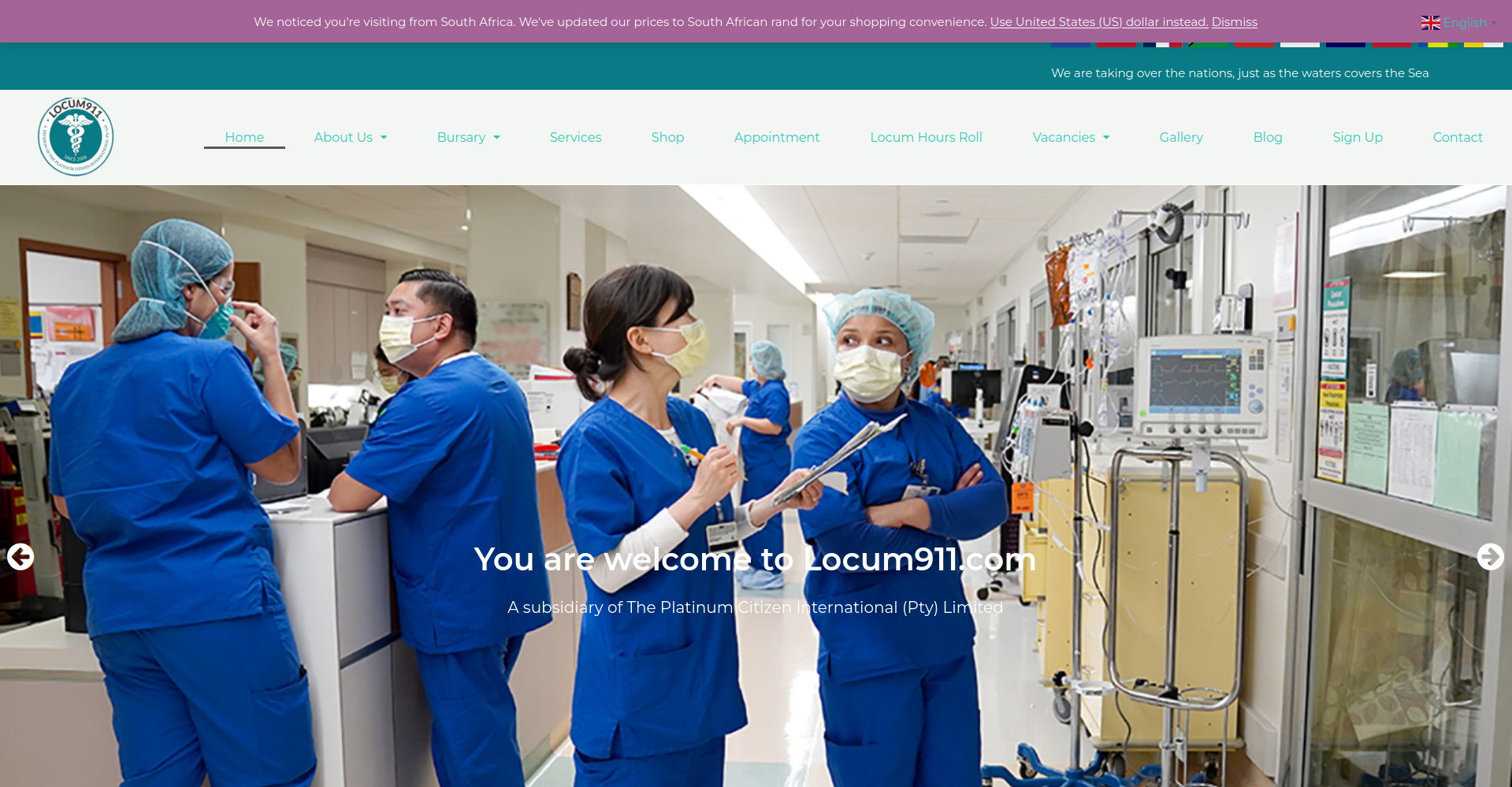In the image, four nurses are engaged in conversation, clearly indicating a healthcare setting such as a hospital or clinic. All the nurses are wearing blue scrubs, a common uniform in medical environments. The nurse in the center front is particularly detailed; she is wearing a white long-sleeve shirt underneath her scrubs, and her ID badge, which features a small panda clip on the chain, is flipped backwards. She is donning a pale yellow mask, and her brunette hair is styled in a low bun with swooped bangs toward the right side of her face.

To her right is another nurse who appears to be Hispanic. She is also wearing a mask, which could be either pale yellow or white, and a light blue hairnet. Her ID badge seems to be facing forward but is obscured by her crossed arms.

To the right of this nurse is a medical device, potentially an EKG or vital signs monitor. The machine has an off-white border, gray controls at the bottom, and several light blue buttons. The screen shows various lines, indicative of a recent EKG reading. The top and bottom of the screen are bordered with light blue strips.

In the background, another woman can be seen lifting what appears to be a stack of paper towels. She is wearing protective shoe covers, commonly known as booties, which are light blue in color.

The central text on the image reads "You are welcome to locum911.com," followed by smaller white lettering that states, "A subsidiary of Platinum Citizen International (PTY Limited)."